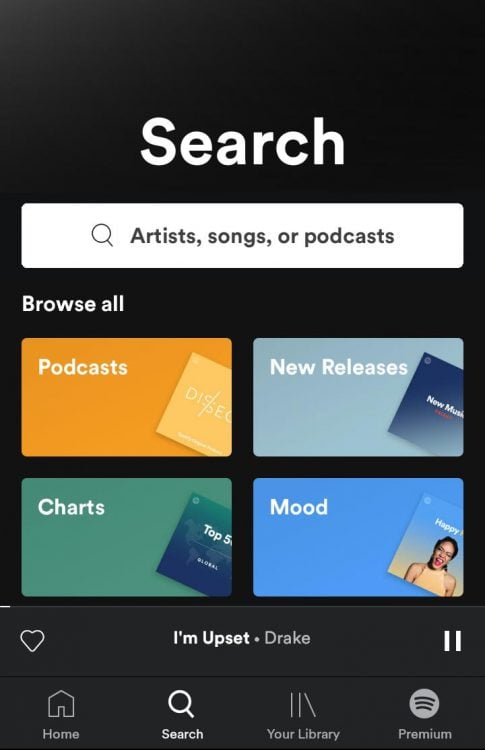This image features a digital interface on a black background. At the top center, bold white letters spell out "Search," with a white search bar just below. Inside the search bar, there is an icon that resembles an hourglass or magnifying glass, and the text within the bar reads "Artists, songs, podcasts" in black. 

Beneath the search bar, aligned to the left, the text "Browse all" appears in white. Occupying the space under this title are four colored boxes arranged in a grid, two on the left and two on the right. The top-left box is orange and labeled "Podcasts" in white. To its right, the top-right box is blue, marked "New Releases." The bottom-left box is green with the word "Charts" in white at the top. Finally, the bottom-right box is a darker shade of blue and labeled "Mood" in the upper-left corner in white.

Below this section are two black horizontal bars that span the width of the page. The top bar features a white heart outline on the left, followed by the text "I'm Upset - Drake" in the center, and a pause button (two vertical white lines) on the right.

At the very bottom of the image is a navigation bar with four icons. From left to right: a home icon with "Home" written underneath, a magnifying glass icon with "Search" below, a library icon consisting of two lines with a third leaning against the middle line, labeled "Your Library," and finally, a white circle containing three horizontal bars, stacked, with "Premium" beneath it.